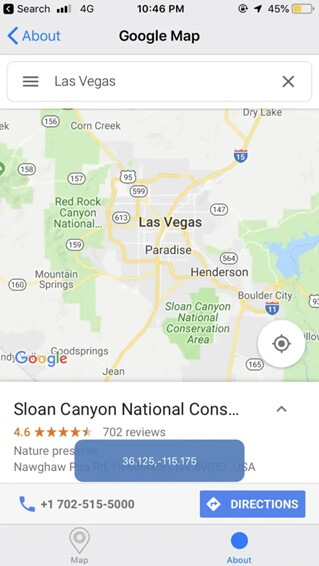The image is a screenshot of a mobile device displaying a Google Maps search result for Las Vegas. At the top of the screen, the device shows essential status indicators: the time is 10:46 p.m., the network signal strength is four out of five bars, the mobile network is 4G, and the battery level is at 45%. The UI is set against a gray background, with the word "About" appearing below the status bar.

Central to the image is the Google Maps interface showing a zoomed-out view of the Las Vegas area. Prominent nearby landmarks are clearly visible: Red Rock Canyon National Conservation Area to the left, Sloan Canyon National Conservation Area below, and an unlabeled green space featuring a lake to the right.

Beneath the map, details about Sloan Canyon National Conservation Area are highlighted. It has received a rating of 4.6 stars from 702 reviews. These details are partially overlaid by a blue box containing geographic coordinates (36.125, -116.175), which possibly represent the latitude and longitude of the location. Additionally, a phone number for further inquiries and an option to get directions to Sloan Canyon National Conservation Area are also visible.